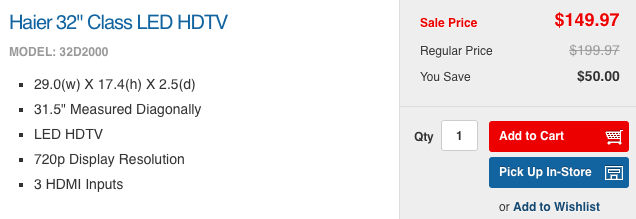This screenshot showcases the product details and sales information for a 32-inch class LED HD TV by Haier. The left side of the image features a white background with "Haier" written in blue letters at the top. Below it, the model number "32D-2000" is displayed in light gray. The specifications are listed as follows:

- Dimensions: 29.0" (W) x 17.4" (H) x 2.5" (D)
- Screen size: 31.5 inches (measured diagonally)
- Type: LED HD TV
- Display resolution: 720p
- Inputs: Three HDMI inputs

On the right side of the screenshot, there is a gray box detailing the sales information. The sale price is prominently shown in red as $149.97, with the regular price of $199.97 crossed out in light gray. The box also notes the savings of $50. Below this, a quantity selector is present alongside a red "Add to Cart" button. Further options include a blue "Pick Up in Store" button with a storefront icon and an "Add to Wish List" link.